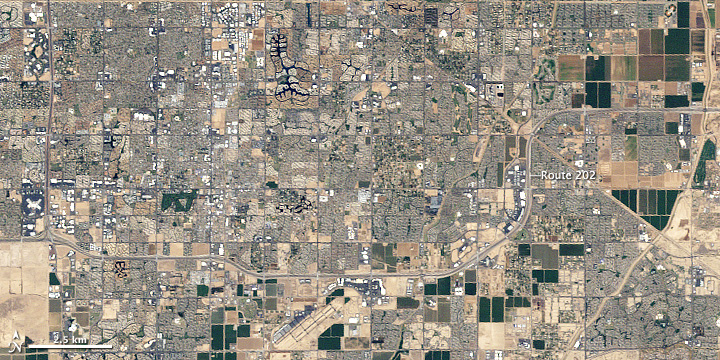This image is an aerial shot of a city, showcasing a detailed satellite map characterized by a palette of browns, tans, whites, blacks, and a touch of gray. Dominating the center is Route 202, a prominent highway that cuts through the urban landscape. The bottom left corner features a scale bar marked "2.5 KM", providing a sense of distance and area coverage. The right-hand side of the image includes text indicating Route 202, emphasizing its significance in the layout. 

In the foreground, the cityscape reveals a mixture of closely packed houses and various buildings, hinting at a residential zone with standard block formations. The landscape is speckled with different land formations and what appear to be dirt patches, suggesting dry, possibly desert-like conditions in some areas. The roadways are distinctly visible, defining the structural grid of the city.

Towards the top right corner, the map transitions into expansive farmland, a stark contrast to the urban density below. The map also includes a key with an arrow marked "North," ensuring proper orientation of the image. Overall, the detailed satellite photo captures a mix of urban and rural elements, road networks, and varied topography, likely sourced from a digital or web-based geographical interface.